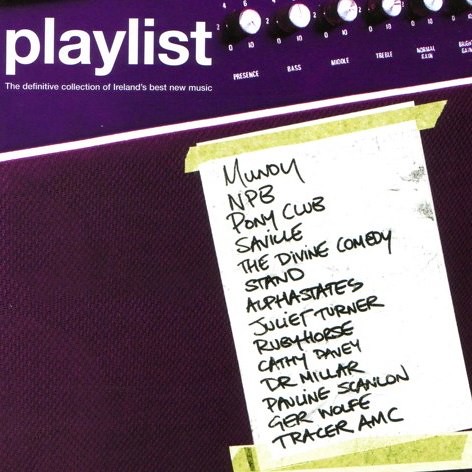The image is a detailed screenshot of a media interface that displays a playlist titled "Definitive Collection of Ireland's Best New Music." The upper section features the large text "playlist" in white, set against a solid black background. Below this, against a white background, is the subtitle "the definitive collection of Ireland's best new music." Central to the image is the playlist itself, consisting of names of various artists and bands, including Stand, Juliet Turner, Ruby Horse, Mundy, NPB, Pony Club, Savile, The Divine Comedy, Alpha States, Kathy Davey, Dr. Miller, Pauline Scanlan, Gare Wharf, Tracer, and AMC. Over on the right side of the image, the interface shows a series of five dials labeled with terms such as "presence," "bass," "mode," and "treble," resembling the controls on a media player. The background has a dark purple hue, resembling carpeted material, providing a contrast to the white and black text of the playlist.